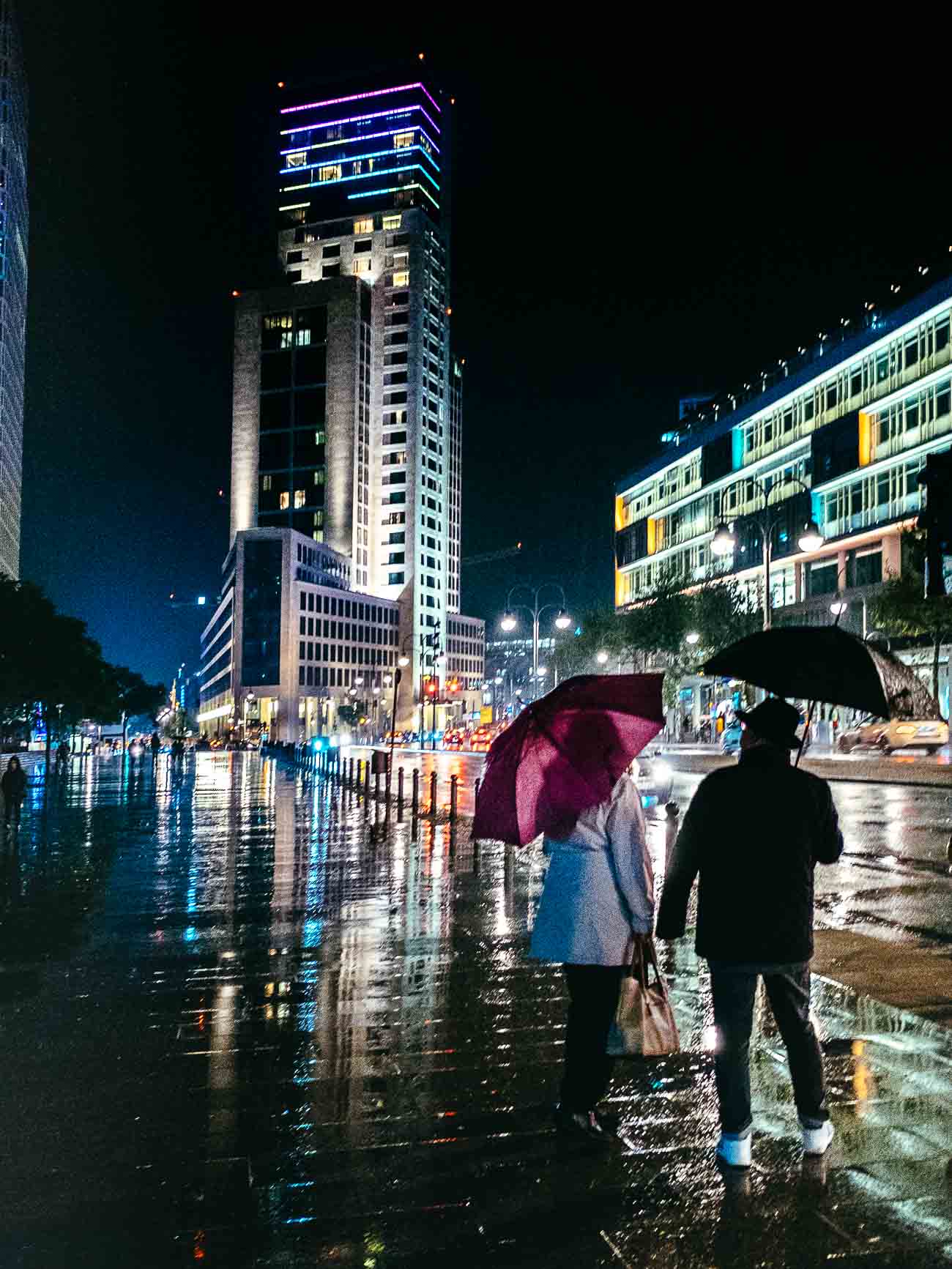A captivating scene unfolds in this nighttime cityscape captured amidst light urban rain. Dominated by the backdrop of a towering skyscraper, the picture exhibits a beautifully lit-up street that reflects off the wet sidewalk and road. The dark night sky adds a stark contrast to the vibrant illumination of the buildings, which vary in height and design. 

In the foreground, two individuals with their backs to the camera walk along the rain-slicked sidewalk, each shielding themselves with umbrellas—one black and the other pink. The man, dressed in white shoes, black pants, a black jacket, and a black hat, holds a black umbrella. Beside him is a woman holding a pink umbrella, clad in a white jacket, black slacks, and carrying a brown purse. 

A three-story hotel with brightly lit windows stands to the right, while a mixture of other buildings, including a prominent 20-story structure, stretches up towards the sky. The reflection of the city's lights shimmers off the rain-soaked ground. Trees line the left side of the scene, adding a touch of nature to the urban landscape. The scene is further embellished by a wide plaza and strategically placed streetlights, lending an almost serene feel to the bustling, rain-drenched city night.